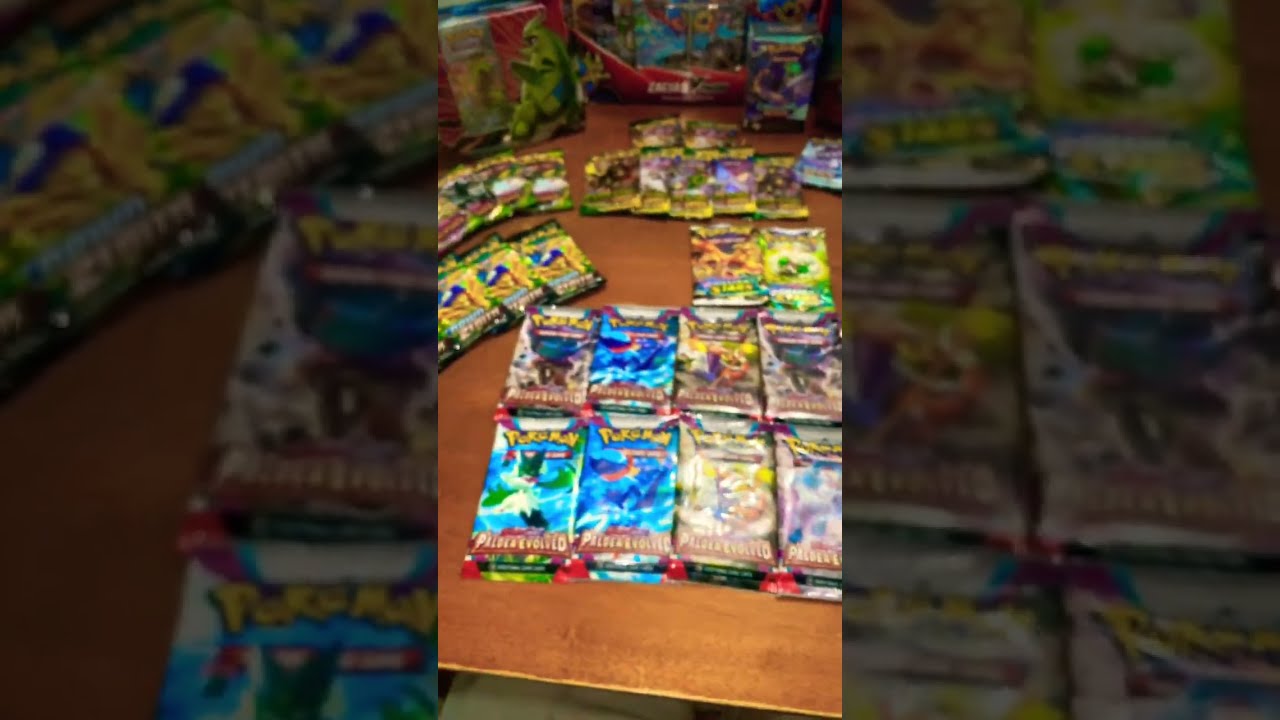The image features a central brown wooden table that stands prominently in the middle of the frame, with a small glimpse of a tiled floor partially visible at the bottom. Sprawled across the table are numerous unopened packs of Pokemon cards arranged in various configurations, including a four by two grid in the foreground, a pair of packs further up, and a row of five above those. In the upper left corner, we see a row of three packs extending off-camera, with another row of three directly above. The packs are vibrantly colored with shades of green, blue, yellow, red, orange, purple, light blue, tan, and white, and their shiny, foil packaging has a noticeable glare that makes some details difficult to discern. Among these packs, the word "Pokemon" prominently stands out as the only readable text. In the background, there are several blurry boxes, potentially also containing Pokemon cards, adding context to the scene suggesting it might be set inside a card collector's store. A close-up of the central image remains sharp while the periphery fades into a soft blur. One notable detail is an identifiable image of Tyranitar, a large green Pokemon, on one of the packs or boxes, adding a specific point of interest within the chaotic display.